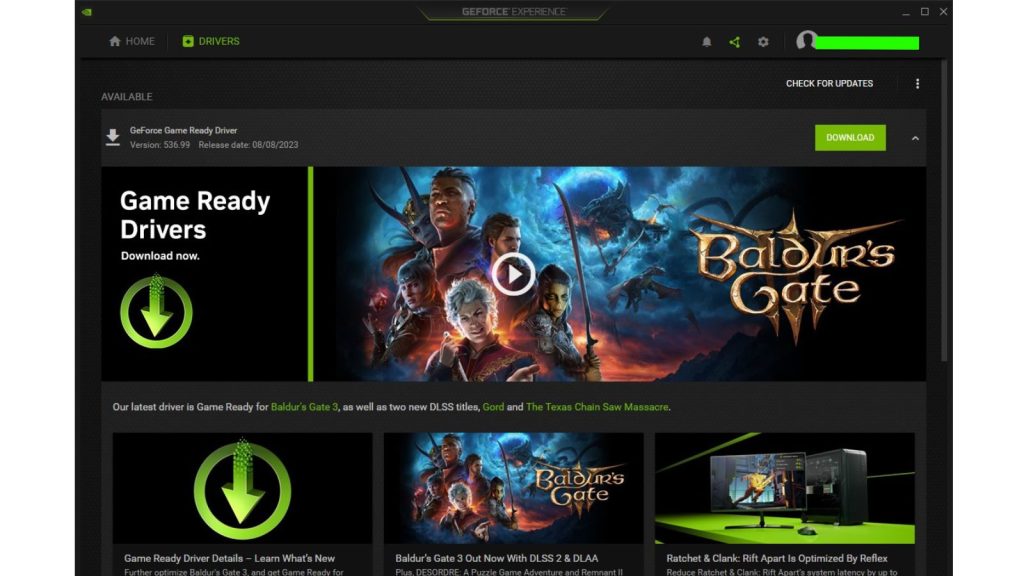The image showcases the interface of the GeForce Experience application, characterized by a sleek, dark grayish-black to green color scheme. At the top of the interface, the title "GeForce Experience" is prominently displayed. In the top left corner, there is a home icon labeled "Home," followed by options for "Drivers."

On the top right, there is a notification bell, which appears triangular in shape, along with settings and control buttons for maximizing, minimizing, and closing the window. The center of the interface highlights a prompt that reads "Game Ready Drivers - Download Now," with an announcement for the game "Baldur's Gate 3" immediately below.

The image features several character renderings: three human characters, an orc-like character with green skin, a black character, and a bluish-skinned female character. Another figure is partially visible in the background, adding depth to the scene. Text below this illustration informs viewers that the latest drivers are optimized for "Baldur's Gate 3" and introduces two new DLSS titles: "Grodd" and "The Texas Chainsaw Massacre."

In the bottom right corner, there is an icon of a computer setup, featuring a monitor and tower with a visible screen, and a mouse placed beside the monitor.